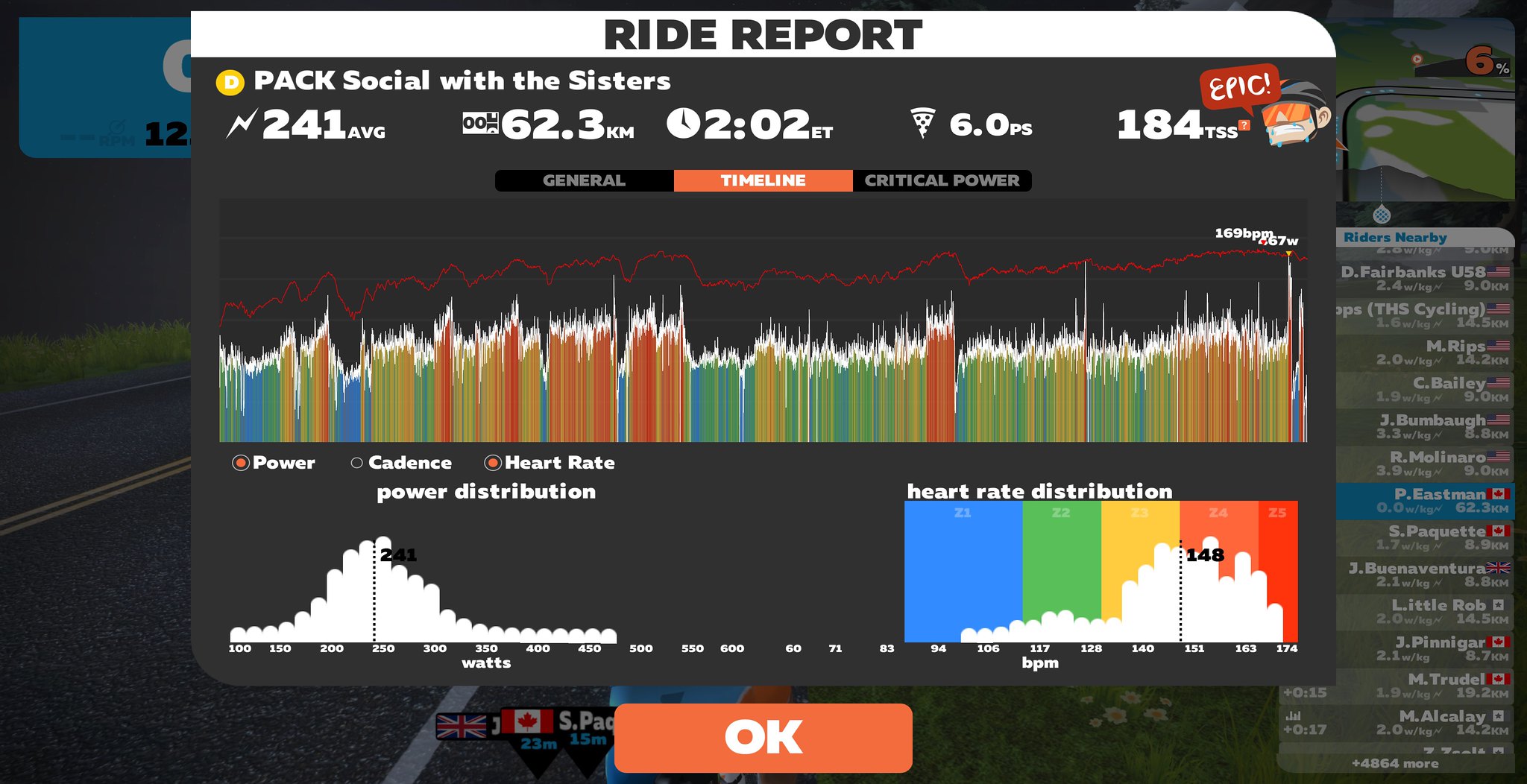The image is a screen capture of a dark-themed web page displaying a detailed ride report window. At the top of the window is a white band with black text that reads, "Ride Report," followed by a black band with white text stating, "PacSocial with the sisters." The report includes various metrics such as "241 average," "62.3 KM," "202 Eastern Time," "60.0 PS," and "184 TSS," all displayed in white text. A multicolored bar graph dominates the center, showing variations in power, cadence, heart rate, and power distribution, with a red line graph overlaying it. 

Below the metrics, there is a small black menu bar with options labeled "General," "Timeline," and "Critical Power," with "Timeline" highlighted in orange. On the right side, there's a heart rate distribution chart, and various other bar graphs with rainbow columns, all contributing to an overall simulation of the ride's data. The interface concludes with an orange "OK" button on the bottom right, standing out in white lettering.